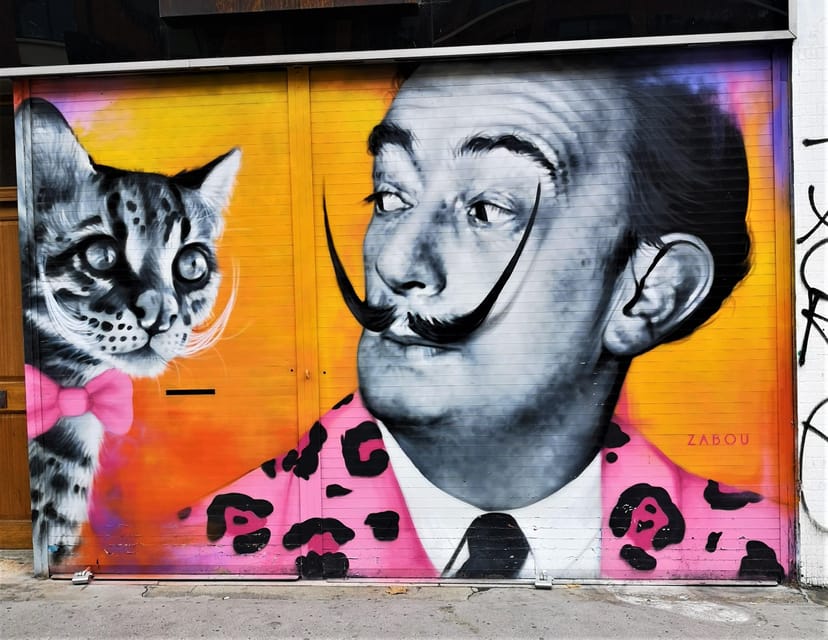The photograph, seemingly taken outdoors, showcases a vibrant and detailed mural painted on what appears to be a large wooden sliding door or possibly a garage/storage door. Central to this mural are two black-and-white figures: a standard house cat on the left, adorned with a pink bow tie, and a man on the right, sporting a pink leopard-spotted suit. Both the cat and the man feature distinctive, upward-curled black mustaches which visually connect them. The background of the mural predominantly consists of bright oranges, with hints of pinks and purples in the top corners, framing the scene. In the bottom part of the image, the visible surroundings include white walls and gray concrete, suggesting an urban setting. There is also text on the wall, "ZABOU," which is likely the artist's signature. This mural blends whimsical and striking visuals, making it a noteworthy piece of street art.